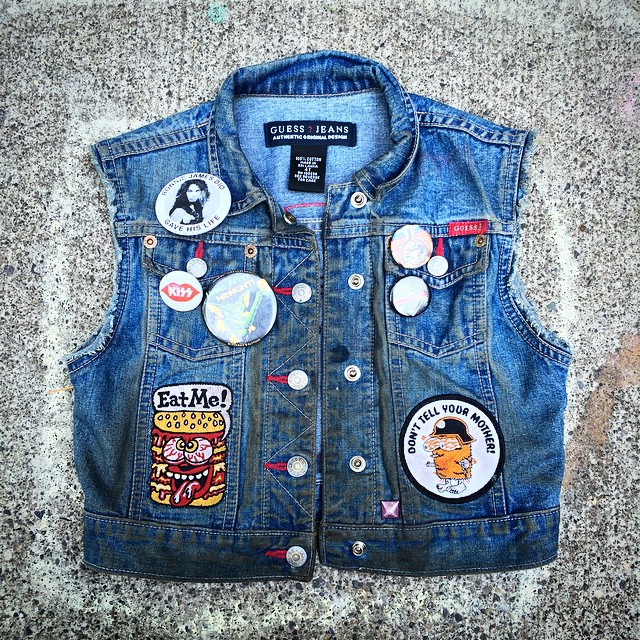This image showcases a distinctive, well-worn Guess Jeans denim vest featuring several notable embellishments against a rough, speckled background of white, black, and gray tones. The vest, with its sleeves cut off, has a black tag at the collar reading "Guess Jeans" in white lettering. The edges of the vest display a combination of red stitching, particularly around the button loops, and silver buttons.

On the left side of the vest, a series of vivid pins and patches are present. Near the top is a pin with a woman's face, followed by a small square pin featuring red lips and the word "Kiss." Below these, a blue and green pin with the word "Midnight" in yellow and a bright flare can be observed. Notably, near the bottom left corner, a grotesquely stylized cartoon burger with bloodshot eyes is accompanied by a speech bubble reading "Eat Me."

On the right side, the vest's lower section features a circular patch displaying a character wearing a black hat and smoking a cigarette, with the phrase "Don't Tell Your Mother" above it. Nearby, the upper right side is marked by a red square logo tag that says "Guess." Additional pins are visible, but due to bright glare, their details are obscured.

Overall, the vest's combination of quirky and edgy embellishments, along with its distressed and personalized appearance, gives it a unique, rebellious charm.